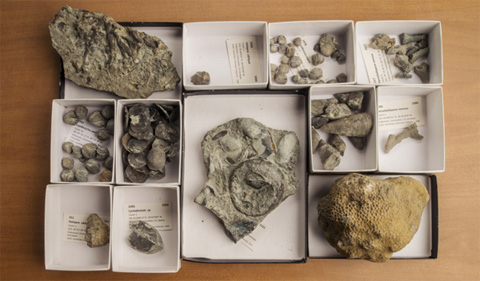This overhead photograph features a meticulously arranged collection of geological specimens and artifacts, housed within twelve small white and black-bordered cardboard boxes, each containing various rocks and fossils. The arrangement forms an approximate rectangular shape, resting on a wooden table visible in the background.

In the top left corner, a large gray rock occupies a white box. Adjacent to it, three more white boxes occupy the top row: the first contains a single rock with an unreadable note, the second houses several small gray rocks, and the third is filled with multiple rocks of varying shapes and sizes.

The middle row includes a prominent black-bordered box with a singular large gray rock, possibly a fossil, with a textured surface indicative of imprints. To the right of this, the two small white boxes contain small gray rocks, with the rightmost box housing a single rock.

The bottom row, starting from the left, showcases four small white boxes. The top two boxes in this formation contain numerous gray rocks, while the bottom two contain one small gray rock each. Additionally, the box positioned at the far bottom right has a distinct brown rock with fossilized markings, surrounded by a black border.

Some specimens extend beyond the edges of their boxes, and several boxes include small cards with inscriptions that are not legible within the photograph. These descriptions suggest a systematic approach to categorizing and identifying the collection, indicative of an archaeological or geological study.